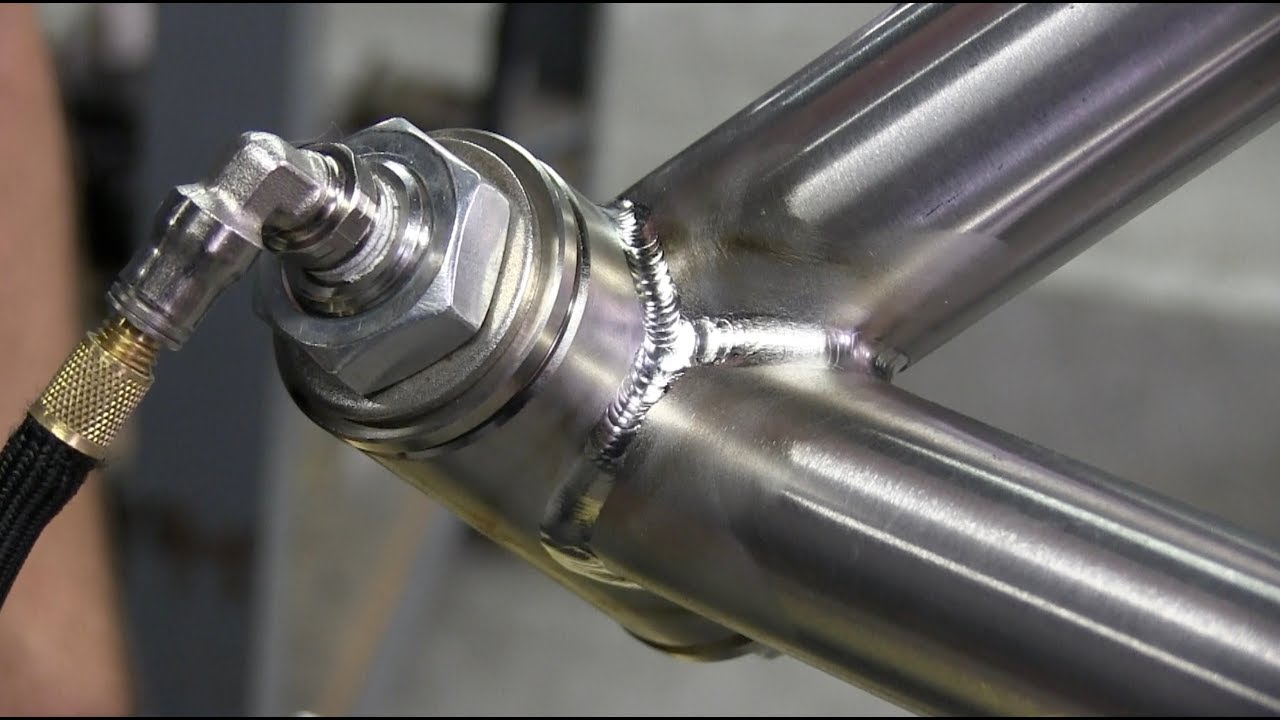This horizontal rectangular image is a close-up view of an industrial metal fixture, prominently featuring two large, likely cast iron pipes. These pipes extend from the lower and upper right-hand corners, forming a V-shape, and converge at a robust valve. Attached to the valve via a tight brass fitting is a black rubber hose, which exits the image to the left and appears secured for functionality. The valve is detailed with a hexagonal nut and several round metal components, including shiny silver and gold connectors that create an intricate assembly. Although the background remains blurry, dominated by shades of gray and some brown, it hints at an industrial environment. The image highlights the strong welds and sturdy construction of the fixture, suggesting it might be used to direct or regulate gases.